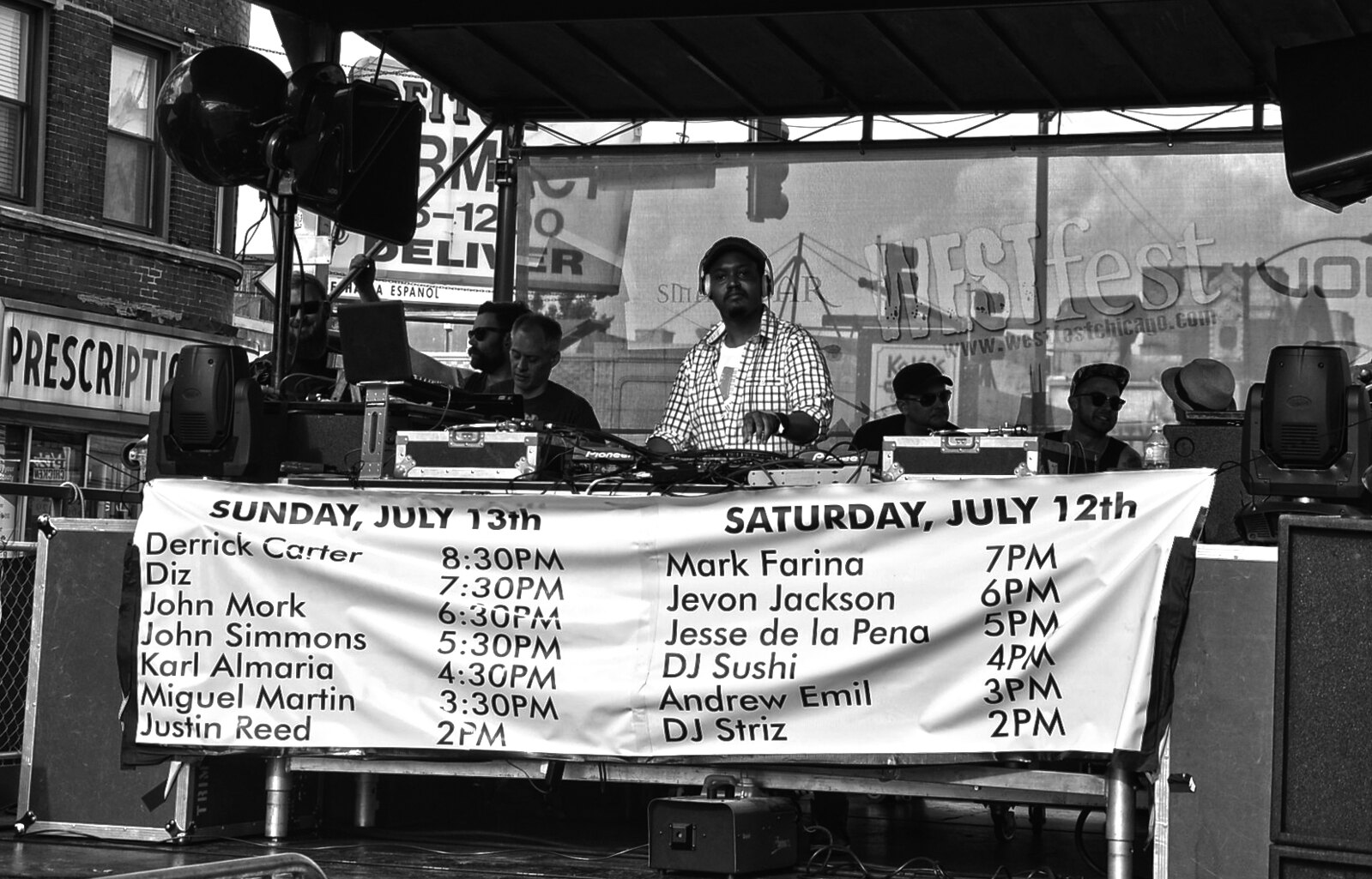In this black-and-white photograph, we have a detailed view of an outdoor DJ performance set on a hard surface stage. The image is in landscape orientation, wider than it is tall, typical of a scenic design. At the center of the stage stands an African American DJ, distinguished by his white and black checkered shirt and over-the-ear headphones, diligently working over a record player. The DJ is surrounded by various sound equipment, creating a hub of musical activity. Flanking him, to his left and right, are several individuals; three men are seated to his right, while two seated and one standing individual are on his left.

Across the front of the stage is a large white banner, split into two sections, each detailing a lineup of performers. The left side of the banner lists names and appearance times for Sunday, July 13th, while the right side follows the same format for Saturday, July 12th. Specific names like Derrick Carter, Diz, John Mork, John Simmons, Carl Almaria, Miguel Martin, Justin Reed are marked for Sunday, and Mark Farina, Javon Jackson, Jesse de la Pena, DJ Sushi, Andrew Emil, DJ Strizz for Saturday, are featured prominently.

In the backdrop, a two-story brick building on the left side displays the word "Prescription," hinting at a pharmacy, with additional signage partially showing "deliver" and a phone number. Overhead, speakers are mounted at the corners of the outdoor roof, which shelters the stage area. Further in the distance, an overhead scrim reads "West Fest" along with the website www.WestFestChicago.com and various sponsor names, highlighting the festival setting of this outdoor concert occurring in the middle of the day.